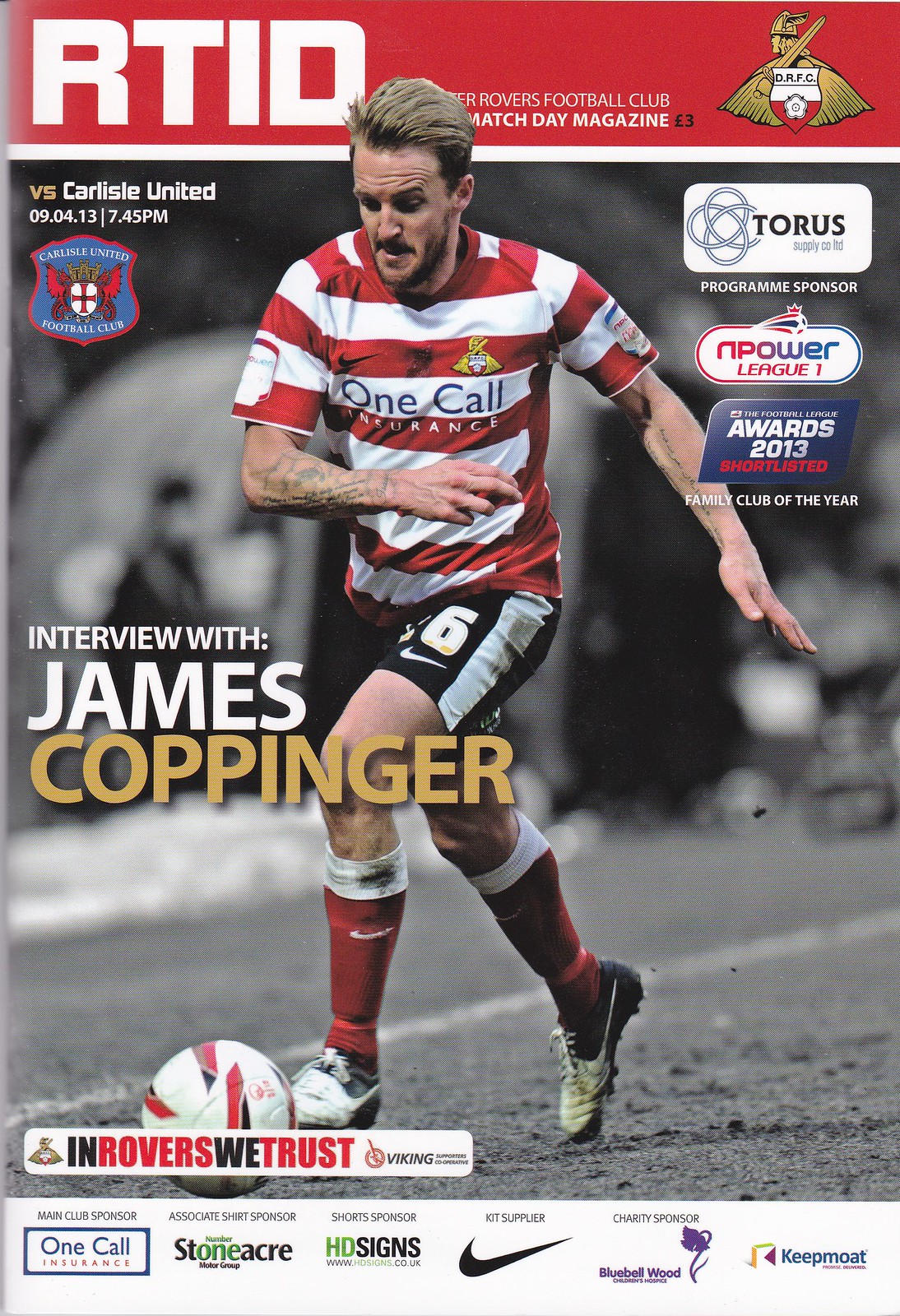The cover of the Match Day magazine for the Doncaster Rovers Football Club prominently features an action shot of James Coppinger kicking a soccer ball. Coppinger wears the iconic red and white Doncaster Rovers jersey, adorned with the club's Viking logo, the Nike swoosh, and the sponsor logo for One Call Insurance. His number 6 shorts also display the Nike swoosh. The background is a stark contrast in black and white, highlighting the colorful player in the foreground.

The magazine's content is introduced at the top with large white letters "RTID," partially obscured by Coppinger's head, followed by "Rovers Football Club Match Day Magazine." To the top right, the text reads: "versus Carlisle United, 09.04.13, 7.45pm," accompanied by the red and white double-eagle logo of Carlisle United Football Club. 

An advertisement for Taurus Supply Company, the program sponsor, is placed in the top right corner alongside the logo for the N-Power League One and the Football League Awards 2013 emblem for "Shortlisted Family Club of the Year." 

Additional details include the bold announcement, "Interview with James Coppinger," written in gold, and the text "In Rovers We Trust" at the bottom part of the image, with "Rovers" and "Trust" highlighted in red. 

The magazine cover also features a white horizontal stripe at the bottom filled with sponsor logos: One Call Insurance (main club sponsor), Stoneacre (associate shirt sponsor), HD Signs (short sponsor), Bluebell Wood (charity supplier), and Keep Moat. Various headings such as "Asian Club Sponsor" and "N-OT Supplier Charity Sponsor" are displayed, emphasizing the contributions of these sponsors.